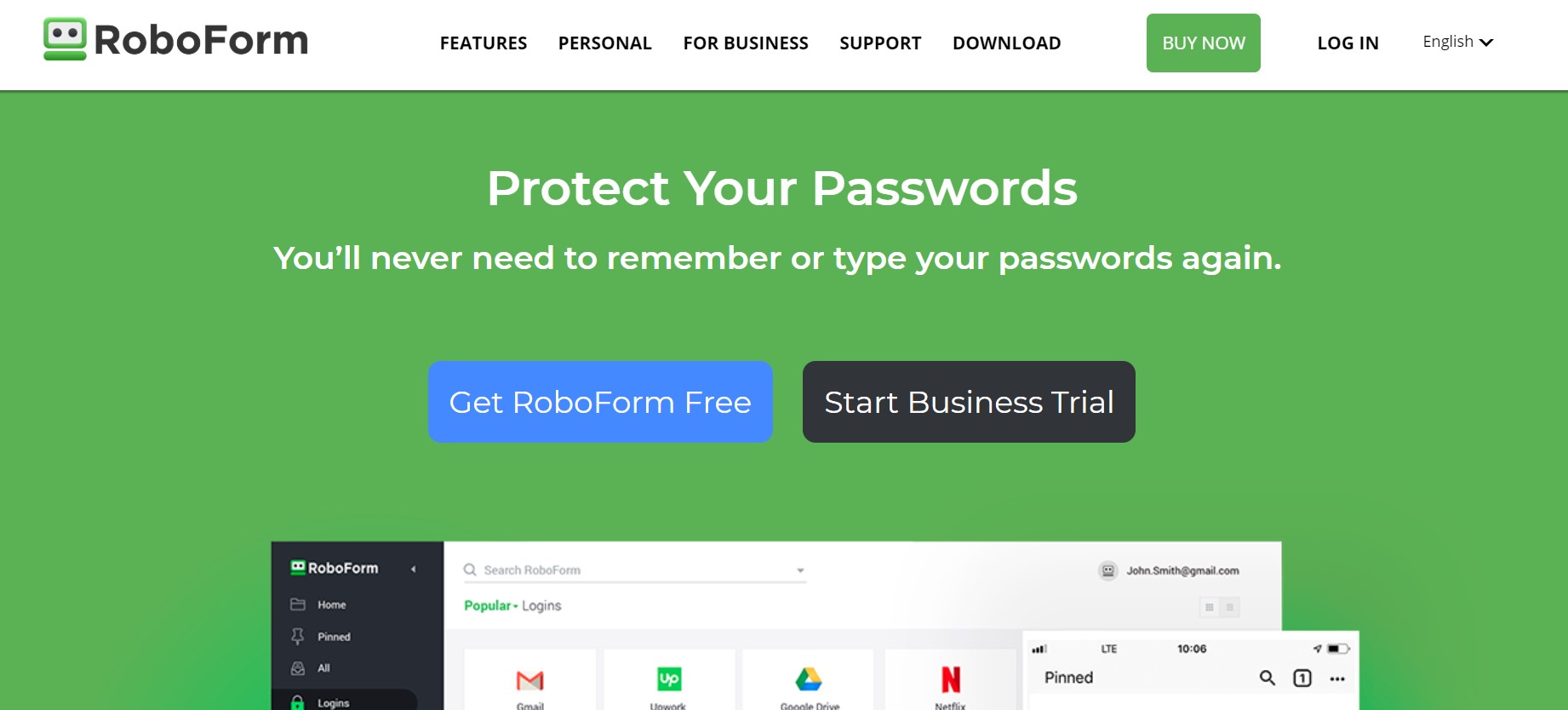This is a detailed description of the RoboForm homepage. On the extreme left, there is a small rectangular green box with two black dots inside it, followed by a bold green line directly underneath. The text "RoboForm" is prominently displayed beside these elements.

The navigation menu includes the following options: Features, Personal, Business, Support, and Download. Below this menu, there is a green button labeled "Buy Now," along with options for logging in and selecting the language, which is currently set to English.

A large green section in the center of the page contains the text "Protect Your Passwords. You'll never need to remember or type your passwords again."

Below this, a blue button invites users to "Get RoboForm Free," and a black button offers a "Start Business Trial" option. The page also features an example illustrating how RoboForm works. The prevalent use of the green color emphasizes the brand's design preference. RoboForm appears to offer free usage for personal accounts and trial options for corporate or business accounts.